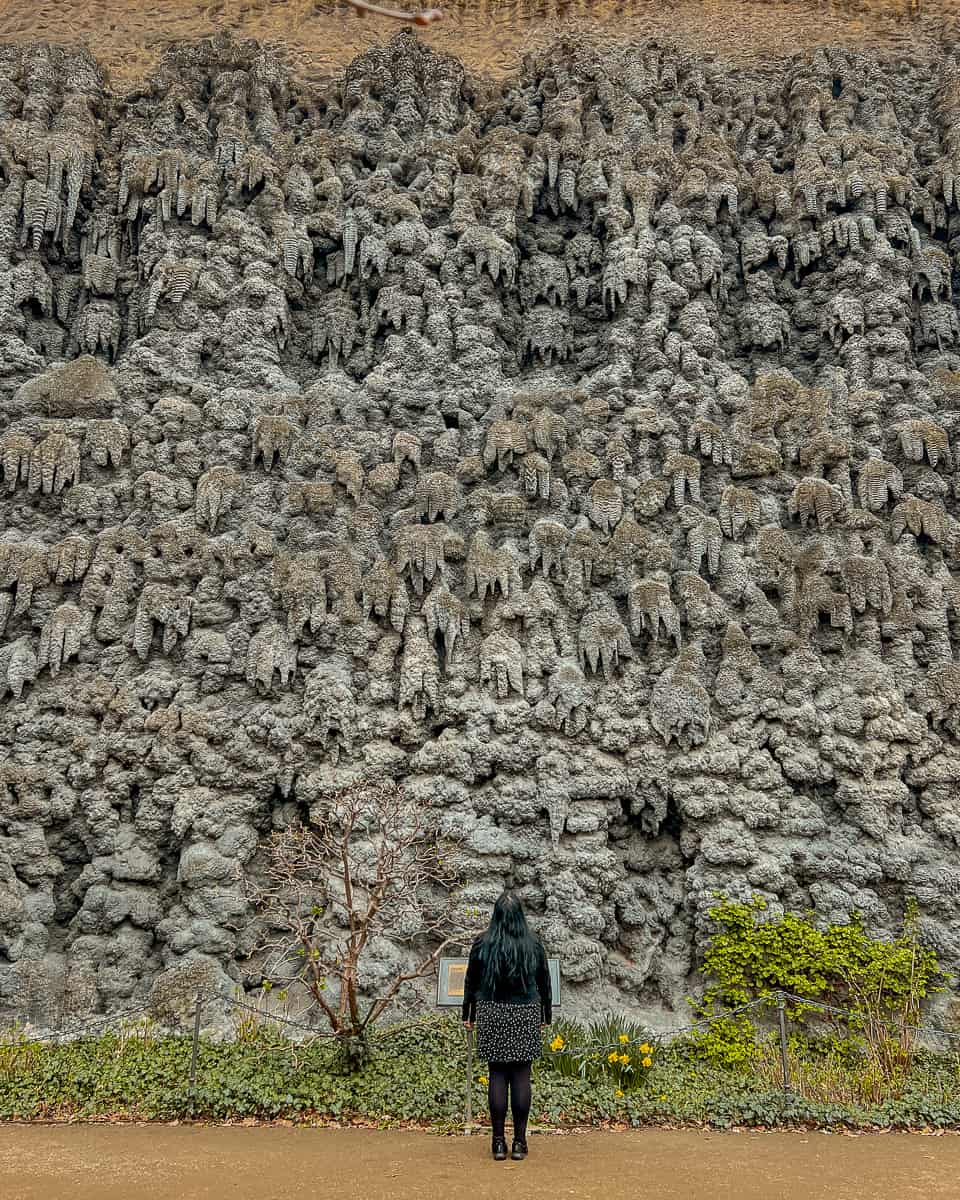In this detailed outdoor image taken during the day, a woman stands on a tan or brown dirt trail with her back to the viewer, gazing up at an imposing, stone-patterned wall or mountain. This wall has intriguing contours resembling petrified flowers or stalactites, with sections of grey and brown hues. The woman is dressed in a black long-sleeve shirt, a black and white spotted vest or skirt, black leggings, and black shoes. Surrounding her on the ground are various plants, including some grass and yellow flowers, and near her are black poles connected by a black chain. A plaque with text, though not legible, is situated in front of her, adding context to the vast and interestingly shaped stone wall she is observing. The overall colors of the scene include grey, brown, shades of green, yellow, silver, and very dark green, with no additional text visible beyond the plaque.